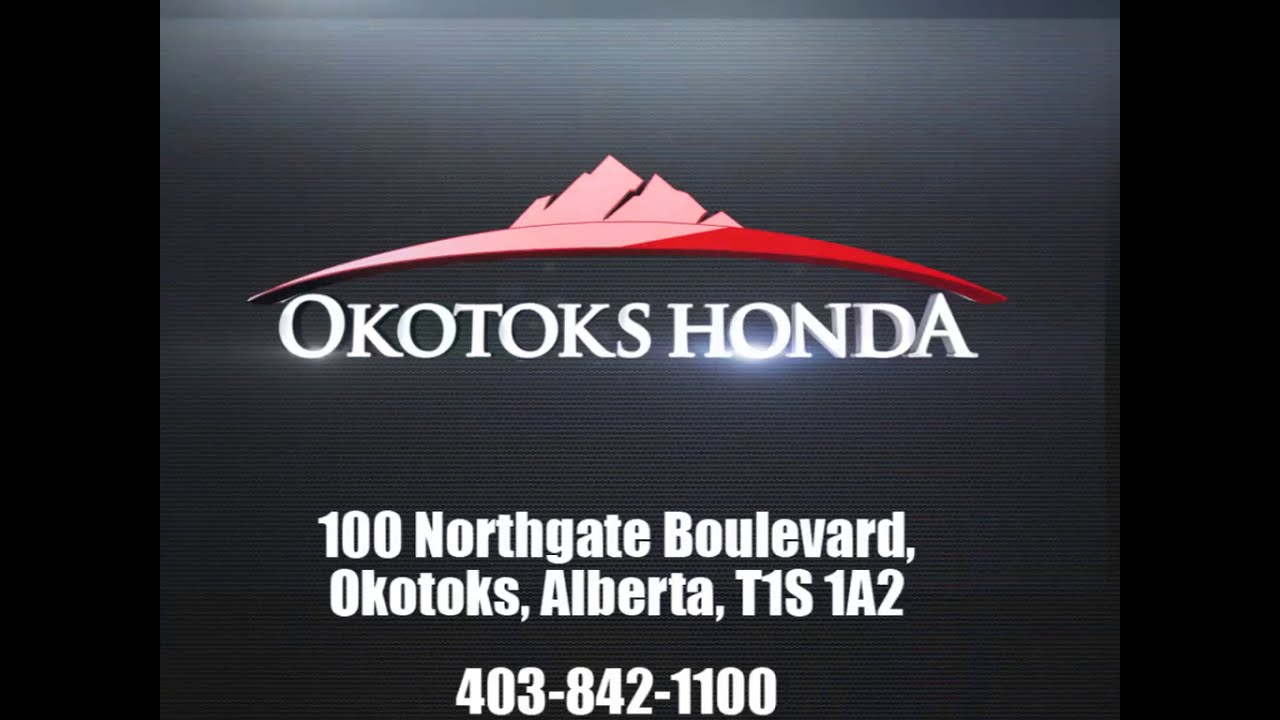This advertisement for Okotoks Honda features a sophisticated color illustration in landscape orientation. The image is framed with vertical black stripes on both the left and right sides. The main content sits against a backdrop that transitions from light gray at the top to dark gray-black at the bottom, creating a subtle gradient effect. 

At the center of the ad, the text "OKOTOKS HONDA" is prominently displayed in all caps, with the first "O" and the last "A" being slightly larger. The "O" in "HONDA" features an illumination filter at its bottom, giving it a glowing effect. Above this text is a convex curved shape resembling the top edge of a globe, with three small pink mountain peaks inside. A pink swash intersects with a red swash from left to right, adding a stylish flair above the logo.

Below the center text, there are three additional lines of information in white font. The first line contains the address "100 Northgate Blvd." Underneath, it reads "Okotoks, Alberta, T1S 1A2," and the final line displays the phone number "403-842-1100." All these elements together create a visually appealing and informative ad for Okotoks Honda, located at 100 Northgate Boulevard, Okotoks, Alberta.